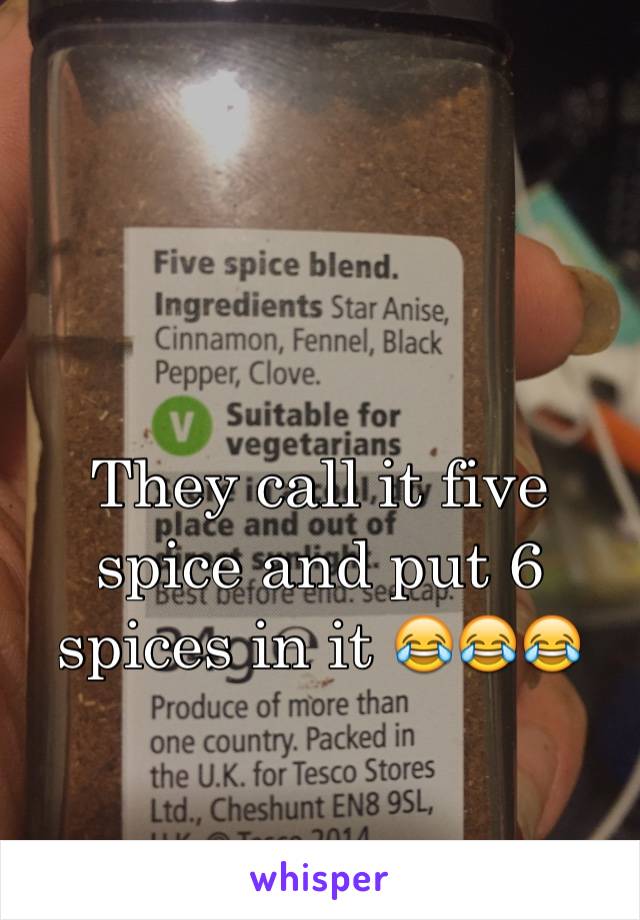This detailed close-up image showcases a plastic or glass bottle containing a brownish powder labeled "Five Spice Blend." The rectangular white label prominently lists ingredients—star anise, cinnamon, fennel, black pepper, and clove—and features a lime green circle with a white "V" indicating it's "suitable for vegetarians." Additional text on the label notes that it's packed in the UK for Tesco. The bottle is held by a person, revealing two fingers with one nail appearing long, suggesting it might be a woman's hand. Superimposed on the photo, large white text humorously states, "They call it five spice and put six spices in it," accompanied by three laughing emojis. Below the image, the word "Whisper" is displayed in lowercase purple font, hinting that this is a meme likely shared on the social media platform Whisper. The object is slightly off-center to the left with blurred background details.